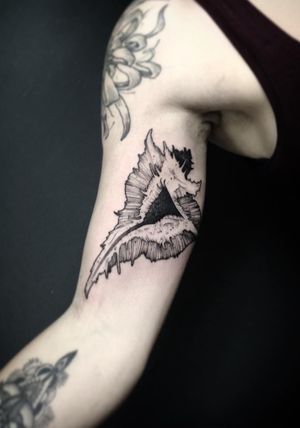This photograph, with a dark gray, nearly black background, showcases the right arm of a person wearing a black tank top. The image has a monochromatic filter, giving the skin a washed-out peach tone. The person's arm is extended towards the lower right corner, partially cut off at the wrist. 

Notable tattoos are visible on the arm: 

- On their shoulder, there is a faded and slightly blurry tattoo resembling a ribbon or a bow.
- The inner bicep features a detailed, dark conch shell design, appearing fresh with clear and pronounced lines.
- On the underside of the forearm, there is a partially blurred tattoo that appears to depict a crown, with a pointed tip at the top and widening out at the base.

The photograph emphasizes the contrast between the newer and older tattoos, enhancing their distinct textures and details against the stark background.